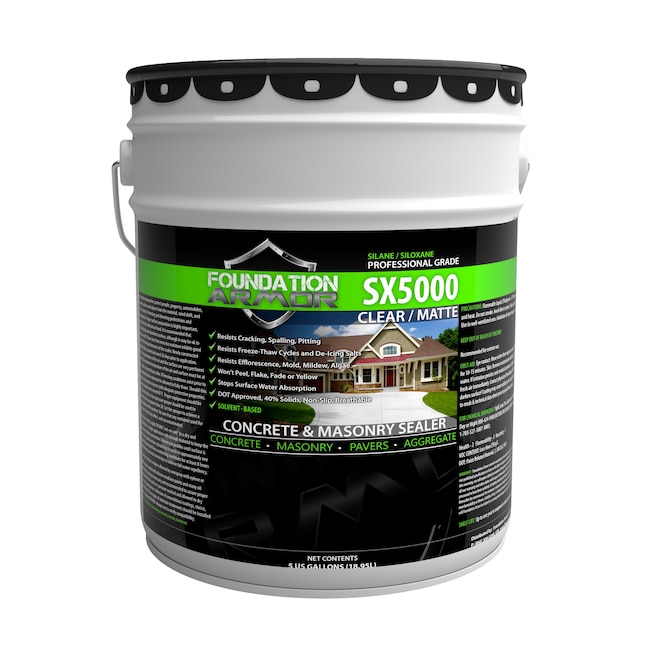This portrait image features a large, white plastic bucket of concrete and masonry sealer with a black lid adorned with small flaps around its edge. The bucket includes a silver handle attached on the left side. The label on the bucket is predominantly black with a bright green stripe that spans horizontally across the center. The label is detailed with multiple pieces of information: starting from the top, there's a silver shield logo over which the green stripe is positioned. The text within the stripe reads "Foundation" in white, followed by "Armor" in silver. Just to the right of this branding, it displays "Professional Grade" in white text, with "Silane Silicone/Siloxane" in green above it. 

Prominently, the label also features "SX-5000" in large white letters. Below this, against the black label, there's an image of a house with a wide white driveway, under which it says "Clear Matte" in white. Continuing down, the label reads "Concrete & Masonry Sealer" and lists "Concrete, Masonry, Pavers, and Aggregate" in green text. The bottom of the label notes the net contents as five U.S. gallons, or 18.951 liters. Additionally, there's a band of white writing in the middle of the label that is not legible, and white text detailing directions on either side, also unreadable in the image.